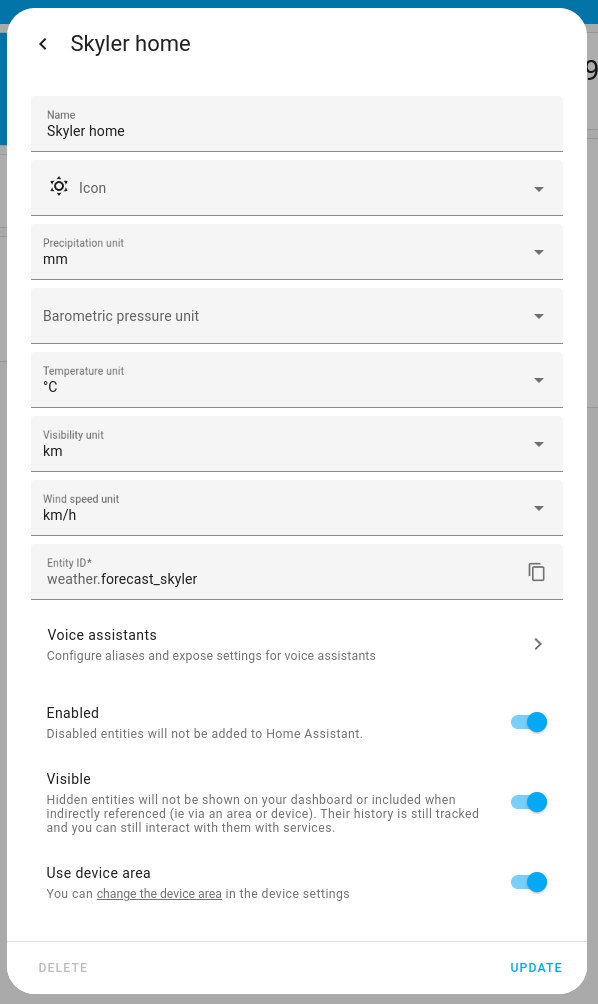Here is a detailed and cleaned-up caption for the image:

---

The image displays a screenshot of the "Skyler Home" configuration interface, featuring a series of light gray rectangular dropdown menus. There are a total of eight dropdown menus, detailing various settings for the Skyler Home weather system. 

1. **Name**: The top rectangle is labeled "Skyler Home."
2. **Icon**: The second dropdown shows a gray sun icon with a downward arrow indicating additional options.
3. **Precipitation Unit**: The third rectangle is labeled "Precipitation Unit," followed by "mm."
4. **Barometric Pressure Unit**: The fourth is labeled "Barometric Pressure Unit."
5. **Temperature Unit**: The fifth rectangle states "Temperature Unit," set to Celsius.
6. **Visibility Unit**: The sixth rectangle is labeled "Visibility Unit," set to kilometers.
7. **Wind Speed Unit**: The seventh identifies "Wind Speed Unit," set to kilometers per hour.
8. **Entity ID**: The last rectangle shows the entity ID as "weather.forecasts_skyler."

Below these dropdown menus are four settings:

- **Voice Assistance**: This section includes options to configure aliases and expose settings for voice assistance.
- **Enabled**: This setting indicates that disabled entities will not be added to Home Assistant; it is currently turned on.
- **Visible**: This setting denotes that hidden entities will not be shown on the dashboard or included when indirectly referenced, but their history is still tracked, and interaction with them via services is possible; it is also turned on.
- **Use Device Area**: This allows for changing the device area within the device settings and is turned on.

The interface also includes "Delete" and "Update" buttons at the bottom left and right corners, respectively.